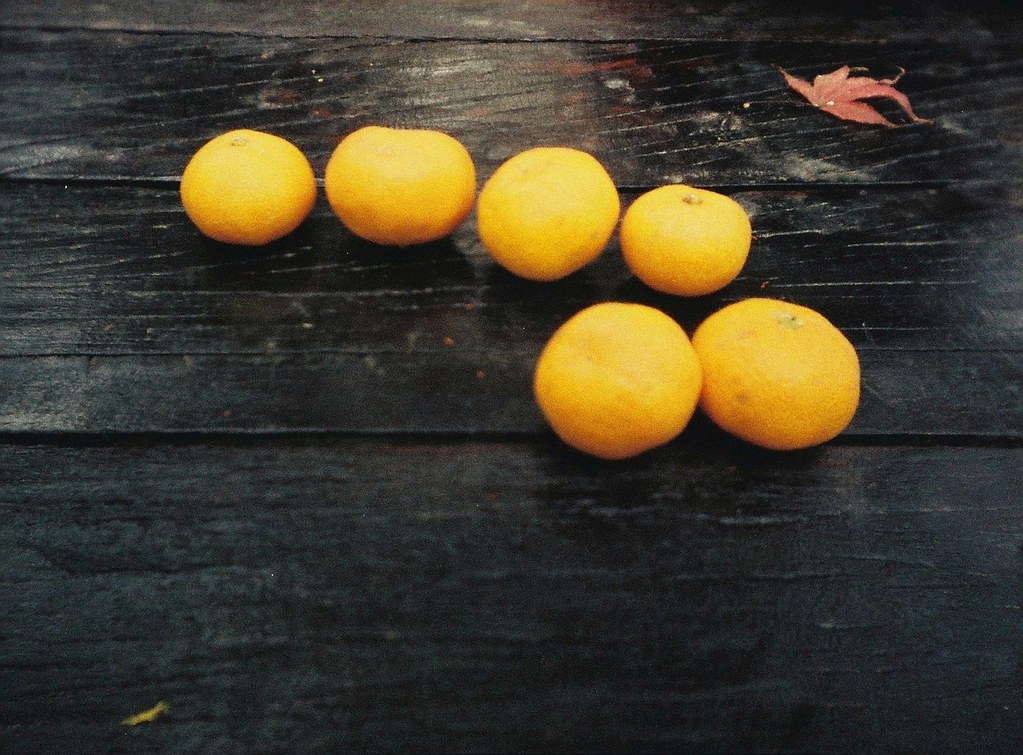This photograph captures six citrus-like fruits arranged on an old, black-stained wooden picnic table. The fruits, which appear more yellow than orange and resemble stubby apples in shape, are positioned in a row of four at the top with a row of two beneath, aligned to the right. Visible on three of the fruits are their stems, while the others showcase their round, slightly dried-out surfaces. The weathered table, featuring four visible slats, exhibits signs of age with dirt, red, white, and gray streaks, and some splitting. There is a sheen on the table from light reflecting off its surface, particularly at the top of the image, and a single red leaf, reminiscent of a maple leaf, lies in the upper right corner.